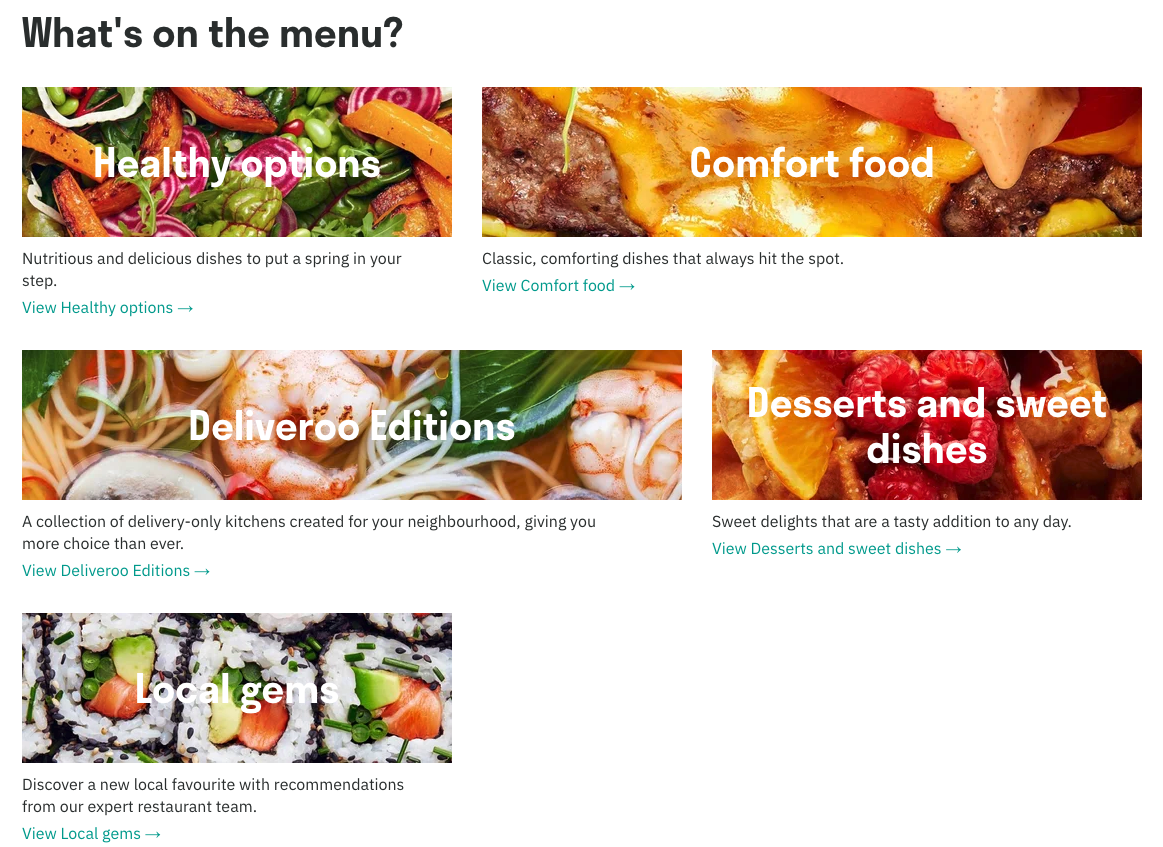The image showcases a vibrant and colorful website menu. At the top, in bold black text, it presents various categories of dishes accompanied by enticing, close-up photographs.

1. **Healthy Options**: The first section highlights vibrant red, orange, and green vegetables, promoting "nutritious and delicious dishes to put a spring in your step." A green button labeled "View Healthy Options" invites users to explore more.

2. **Comfort Food**: The next section features a slightly larger image of a cheeseburger with melting cheese and fresh tomato. It advertises "classic comforting dishes that always hit the spot," with a clickable link "View Comfort Food" to learn more.

3. **Delivery Additions**: This part of the menu showcases a collection of delivery-only kitchens. The image includes an assortment of shrimp, spaghetti, and greens. It offers the promise of "giving you more choice than ever," with a green button "View Delivery Additions" for further exploration.

4. **Desserts and Sweet Dishes**: Featuring glazed fruits such as raspberries and orange slices, this section promises "sweet delights that are a tasteful addition to any day." Users can click on "View Desserts and Sweet Dishes" to satisfy their sweet tooth.

5. **Local Gems**: The final section highlights a colorful sushi platter with white rice and rolled fish and vegetables. It encourages users to "discover new local favorites with recommendations from our expert restaurant team," with a link "View Local Gems" to find out more.

Each section is visually enticing with vivid, close-up imagery that highlights the appeal and quality of the food offered.